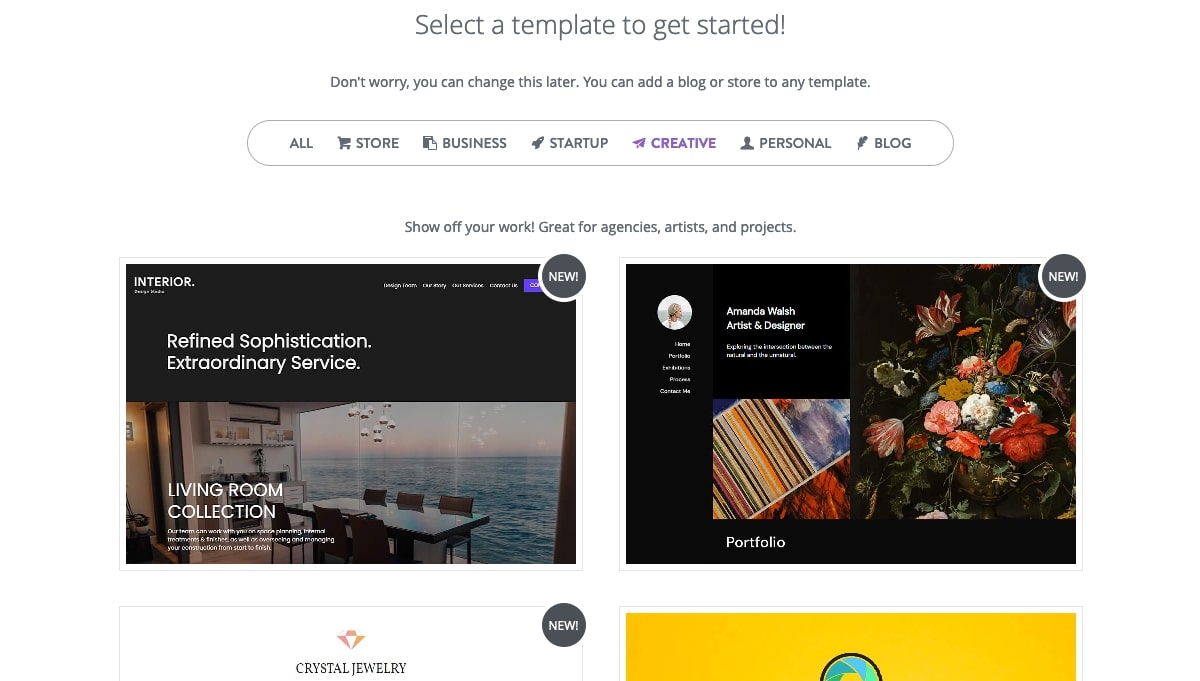This screenshot captures a webpage prompting users to "Select a template to get started." It reassures, "Don't worry, you can change this later," and notes that users can add a blog or store to any template. The template categories displayed include "All," "Store," "Business," "Startup," "Creative," "Personal," and "Blog," with "Creative" highlighted in purple while the others are in black or dark gray text. Below these options, the website encourages users to "Show off your work," ideal for agencies, artists, and personal projects. 

The templates previewed on the page highlight various themes:
1. The first template, titled "Interior," boasts "Refined sophistication, extraordinary service," showcasing what appears to be a living room collection, suitable for a furniture or home decor business.
2. Adjacent to it is "Amanda Walsh," designed for an artist and designer to display her portfolio.
3. Directly below the "Interior" theme is "Crystal Jewelry," which appears to be for a jewelry company, although the full text and images are cut off.
4. To its right is a template with a predominant yellow background, partially showing the top of a ribbon, though the specific details remain unclear.

The webpage serves as a tool for users to build and customize templates for their blogs or websites, offering a creative and personalized way to showcase their work.